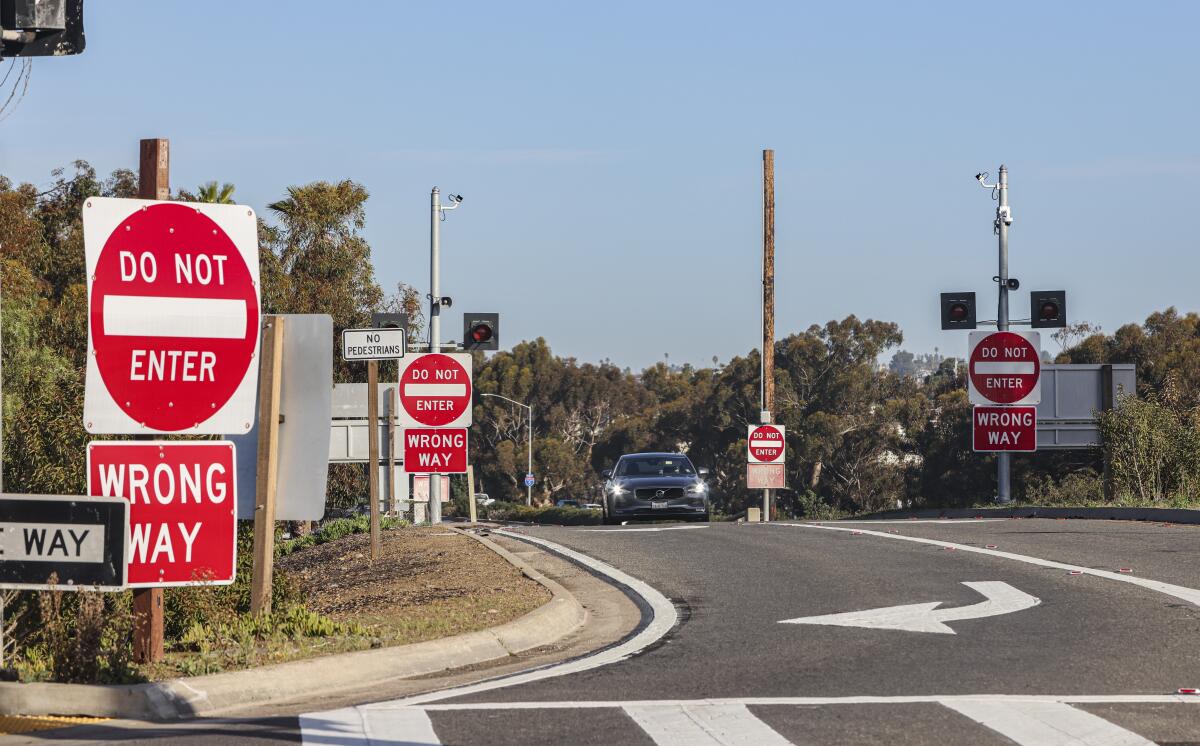The photograph captures a perplexing roadway scene with a turn lane prominently marked by a left-turn arrow on the pavement. Flanking the lane are a total of four 'Do Not Enter' signs—two on either side of the road—augmented by additional 'Wrong Way' signs. Further back, a silver sedan, possibly a coupe, is advancing towards the turn lane, its headlights on as if poised to defy the warning signs. Overhead, surveillance cameras are mounted on the poles that hold the central 'Do Not Enter' signs, while a 'One Way' sign and a 'No Pedestrian' sign add to the mix of conflicting instructions. The background is dotted with pine trees under a clear blue sky, and the scene is anchored by a sidewalk at the bottom of the image. Light posts and what appears to be a railway slat pole are also visible, contributing to the overall sense of confusion.